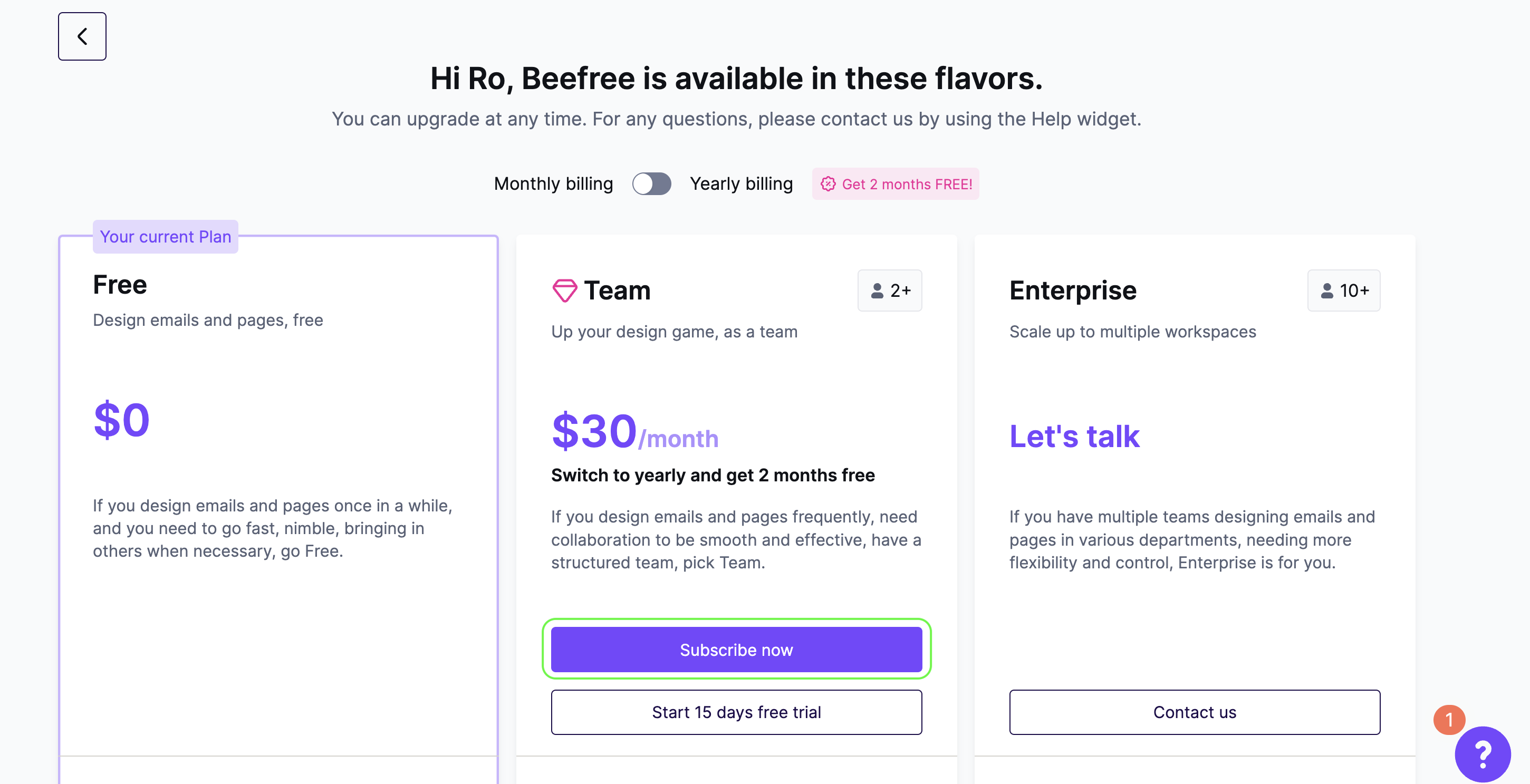This screenshot showcases various subscription plans available through an online platform. At the top, bold black text spells out "HIROBEEFREE" emphasizing the brand's name. The header reads, "HIROBEEFREE is available in these flavors. You can upgrade at any time. For any questions, please contact us by using the help widget."

A toggle switch allows users to alternate between monthly and yearly billing options, accompanied by a pink note that states, "Get two months free." 

The screenshot displays three plans formatted as side-by-side rectangular columns or cards. The first column, labeled "Current Plan," represents the free plan priced at $0. The central column showcases the "Team Plan" designed for groups of two or more people, costing $30 per month. Users opting for yearly billing receive two months free. The final column on the right features the "Enterprise Plan," tailored for teams of ten or more members. 

These options provide various pricing and feature levels to cater to different user needs.